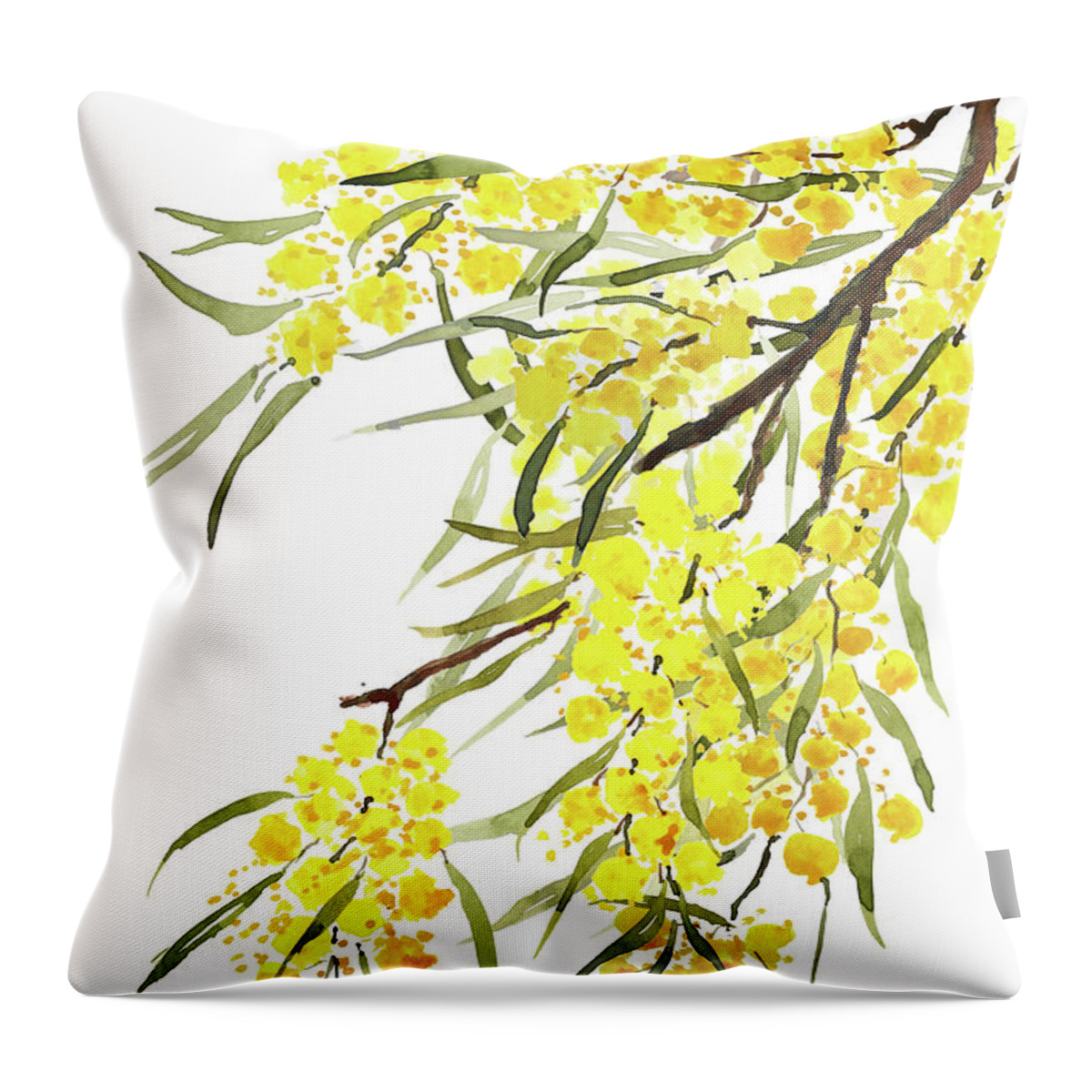In the image, you see a white, square cushion prominently displayed against a white background. The cushion, which has a fluffy, poofy appearance, is clearly a decorative throw pillow. The soft material inside causes the pillow to look slightly cinched rather than perfectly square.

The main design on the pillow is a watercolor painting of a tree branch. The branch is brown and descends from the top right corner toward the center of the pillow. Along this branch, several smaller branches sprout outwards. Delicate, thin olive-green leaves hang from these branches, adding a touch of nature with their faint, light appearance.

Scattered across the pillow's surface are yellow circles resembling flowers. These circles have accents of gold and brown, giving them a contoured look and possibly representing flower anthers. The overall impression is of a branch in the height of bloom, adorned with these soft, yellow blobs that give the illusion of flowers with specks of orange for shading.

The lighting in the image comes from the top right, casting shadows beneath the pillow and to the left side, enhancing the depth and detail of the watercolor design. The pillow stands upright, creating a clear and detailed view of its decorative pattern.